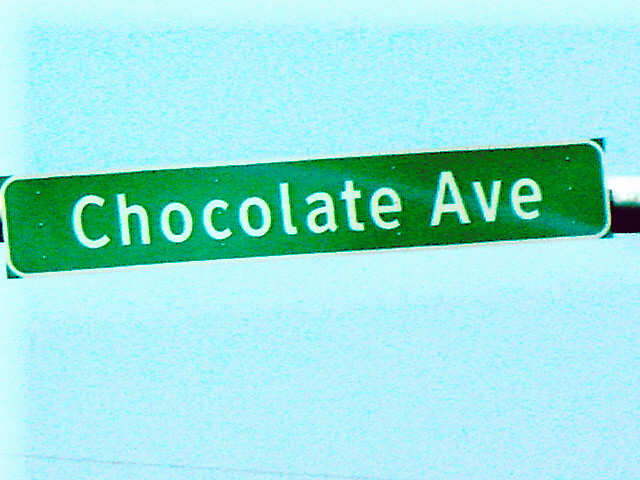The image features a somewhat pixelated photograph with a light blue background. The outer edges of the background appear slightly lighter, forming a subtle rectangular border that is discernibly brighter than the surrounding area. Dominating the center of the image is a rectangular street sign affixed to a black pole. The sign is predominantly green with a smooth, white border lining the edges. Each corner of the sign is accented with distinctive green tips. Bold, white lettering in a clean font spells out "Chocolate Avenue" across the green surface of the sign. The sign is securely fastened to the black pole through rows of screws, arranged neatly in groups of three, running from one end of the sign to the other.